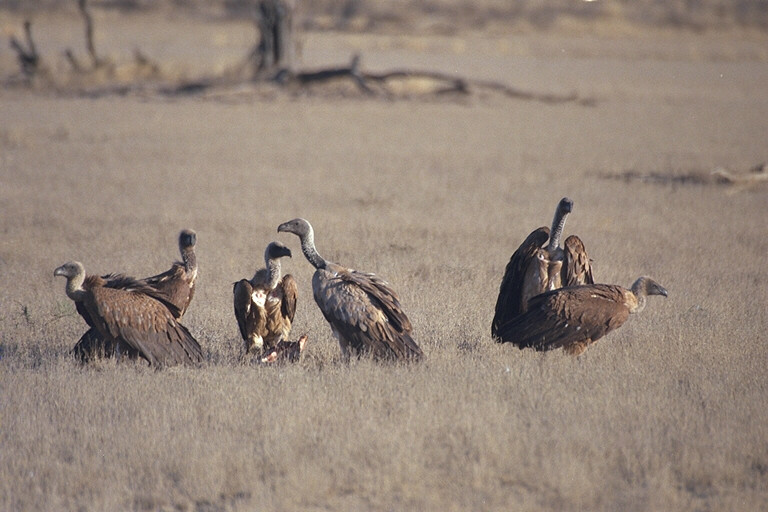In this photograph, we see a group of six vultures huddled together in a vast, brown grassy field. The grass appears to be dead, giving the scene a grayish-brown hue that extends from the bottom to the top of the image. The vultures are large birds with predominantly brown feathers along their backs, contrasted by lighter gray feathers on their necks and chests. Their necks have short, light gray fur, and each bird has a short but sharp dark gray beak. The birds are positioned facing different directions, adding a sense of alertness to the scene. In the background, there are several dead trees with bare, fallen branches scattered on the ground. The scene is bathed in sunlight, which casts a bright light on the birds and the dry field, enhancing the stark, almost monochromatic appearance of the landscape.